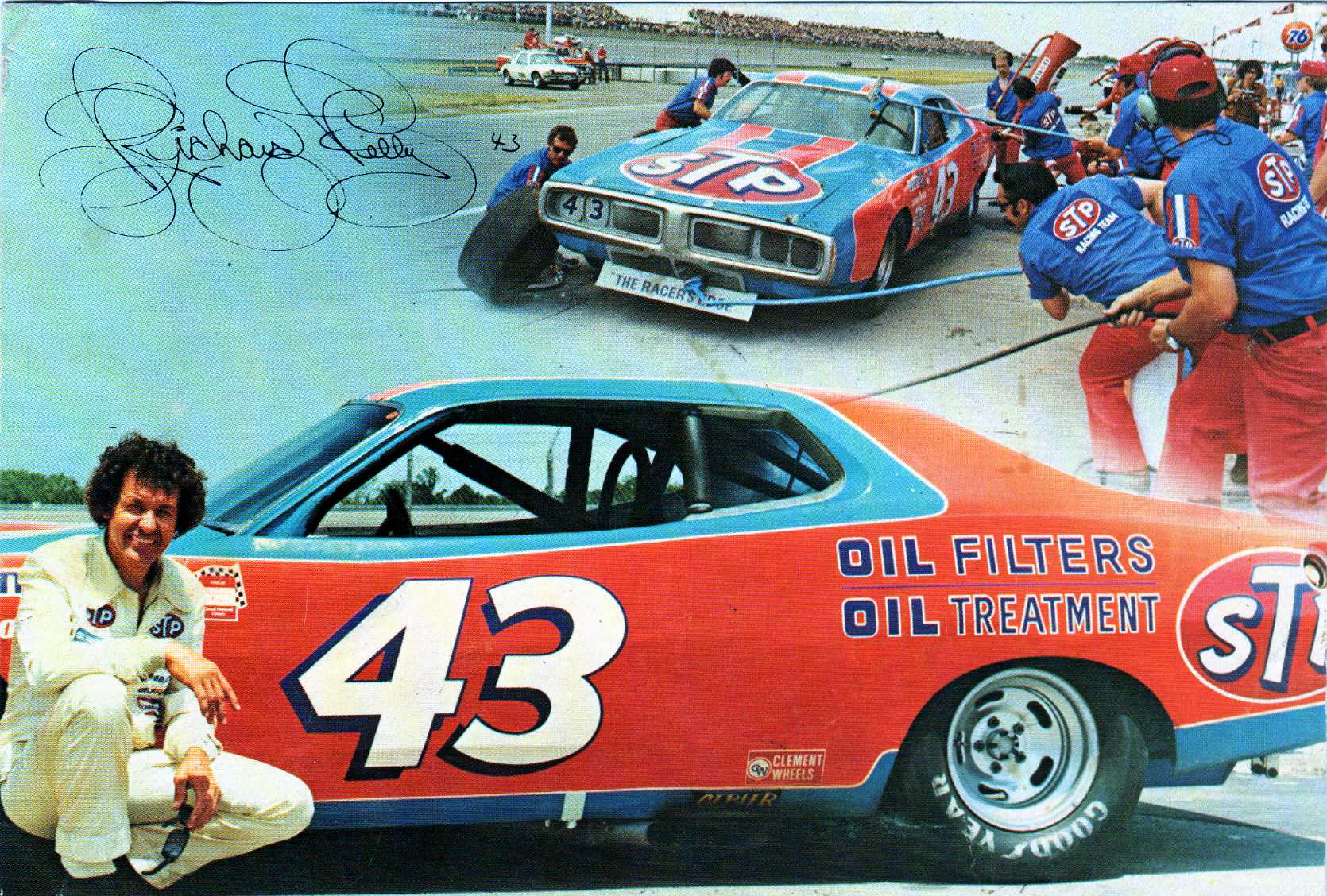The photograph is a detailed montage featuring an orange NASCAR race car with a prominent white number 43 on its sides and blue trim on the hood and top, sporting various logos including "oil filters" and "oil treatment." The top right corner of the montage showcases a pit stop scene, where crew members dressed in blue short-sleeved shirts with red logos and red pants are actively refueling and changing the tires of the race car against the backdrop of an active racetrack with a visible crowd. The top left corner displays a clear blue sky and a cursive autograph, which appears to be signed by Richard Petty, accompanied by the number 43. The bottom half of the image features a man, presumably Richard Petty, in a white racing suit, crouching next to the same race car. The car prominently displays the "STP" logo on the rear bumper and Goodyear tires, adding to the authenticity of the racing scene.